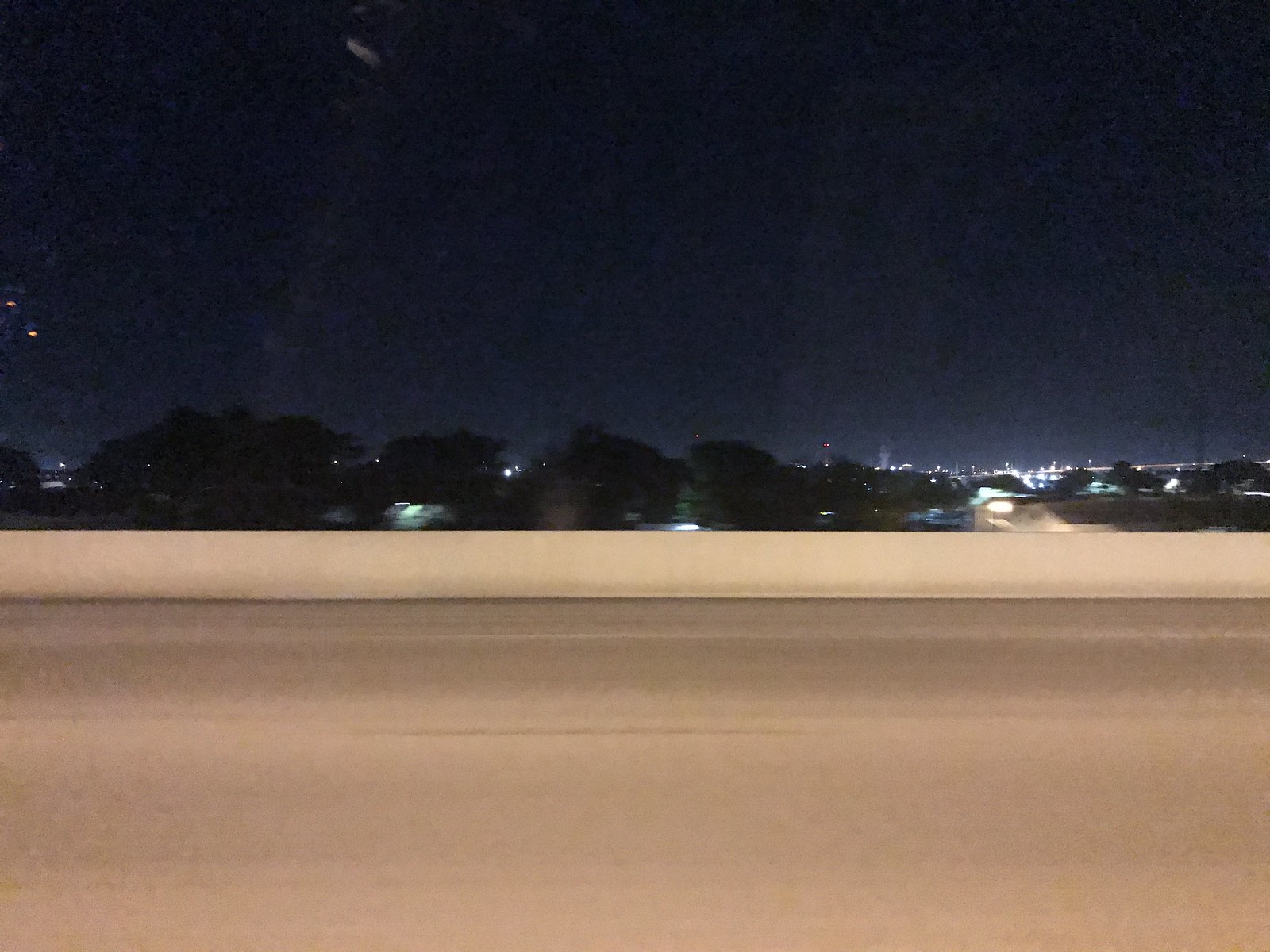A slightly blurry night-time photograph captures a deserted highway from its far side, revealing three lanes of grey pavement. In the distance, a short white concrete barrier separates the highway from a softly glowing cityscape. The sky is a uniform blue, possibly due to light pollution, obscuring any stars. On the left side of the barrier, clusters of green trees are visible, thinning out as they extend to the right. Among the city lights, a white concrete building stands out, illuminated by a bright light from one of its windows.